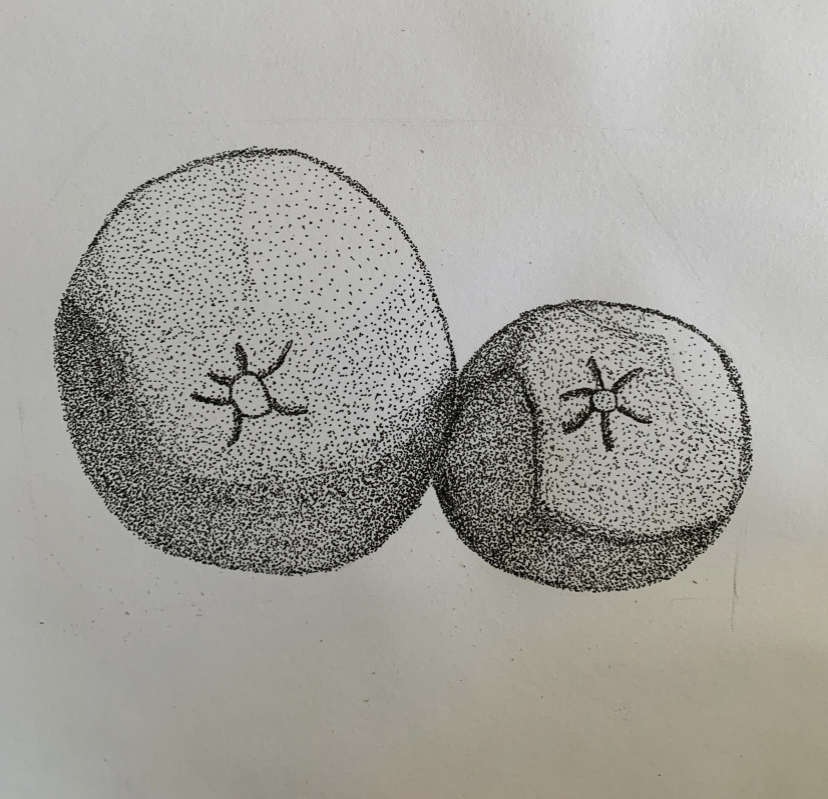This detailed illustration showcases two meticulously drawn oranges on a clean white sheet of paper. The artist employed a pen to create a pointillism effect, using innumerable tiny dots to render the shading, resulting in a textured and dimensional depiction. The orange on the right is larger, featuring a central navel with six distinct, small black squiggles radiating outward. Adjacent to it, the smaller orange—approximately two-thirds the size of the first—exhibits a slightly indented spot on its left side and a smaller navel also adorned with six evenly spaced squiggles. The shading predominantly wraps around the bottom of both oranges, accentuating their curvature and volume. Subtle warping in the paper and faint pencil streaks can be observed, adding a touch of authenticity to the artist's process.